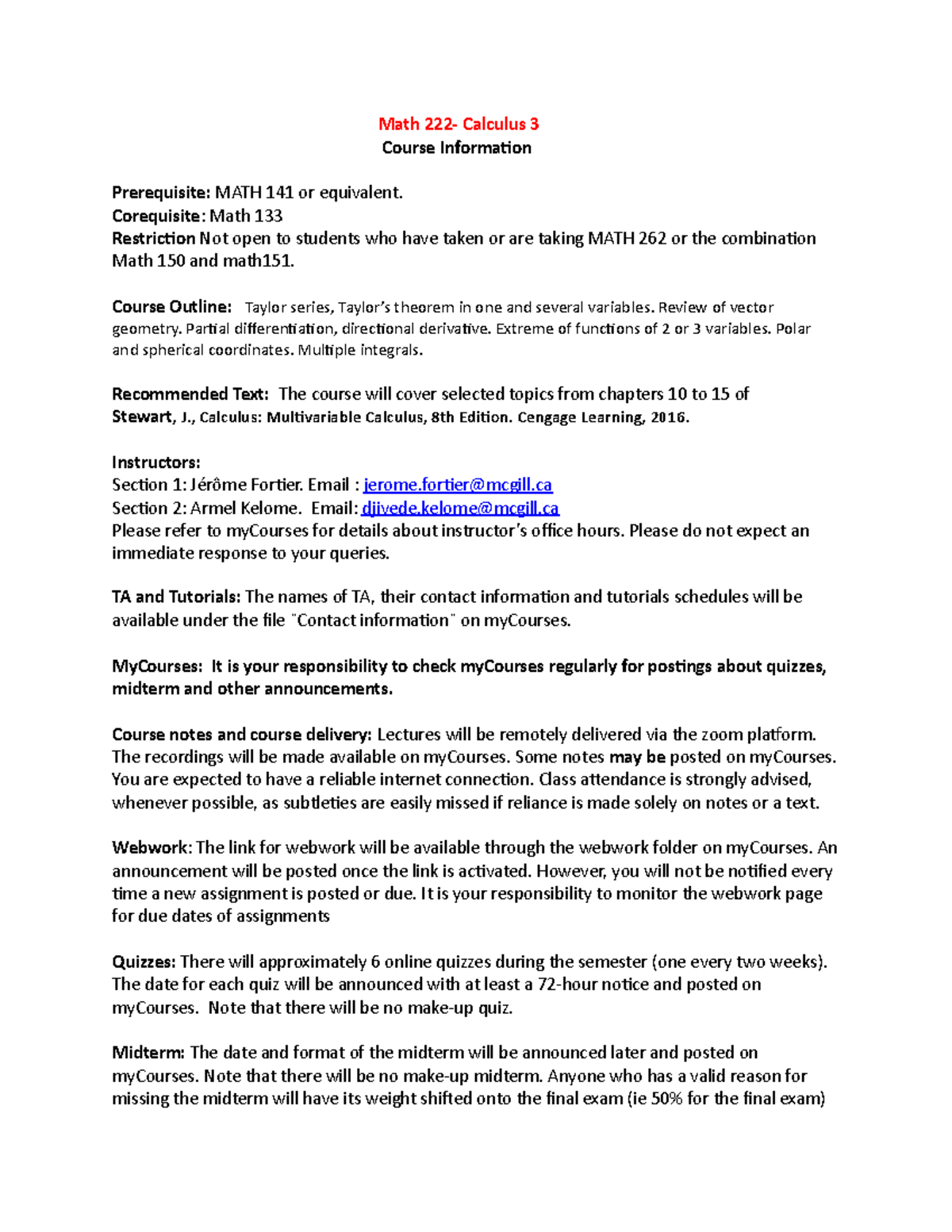**Detailed Descriptive Caption:**

This document is a comprehensive syllabus for "Math 222 - Calculus 3," showcasing detailed course information for a higher-level math class. At the top of the syllabus, prominently highlighted in red text, is the course title, followed by key details in black molded text.

- **Course Information:** 
  - **Prerequisite:** Math 141 or an equivalent course.
  - **Co-requisite:** Math 133.
  - **Restrictions:** Not open to students who have previously taken Math 262 or the combination of Math 150 and Math 151.

- **Course Outline:** 
  The syllabus elaborates on the topics covered, including:
  - Taylor Series
  - Taylor's Theorem in one and several variables
  - Review of vector geometry
  - Partial differentiation
  - Directional derivatives
  - Extremum of functions of two or three variables
  - Polar and spherical coordinates
  - Multiple integrals

- **Instructor Contact Information:**
  - **Section 1:** Taught by Jerome Fortier (Email: jerome.fortier@mcgill.ca)
  - **Section 2:** Taught by Armel Colombe (Email: djiveti.colombe@mcgill.ca)

- **Teaching Assistants (TAs):** 
  - The document directs students to check "MyCourses" regularly for listings of TAs and information regarding quizzes, midterms, and other announcements.

- **Additional Information Sections:**
  - **Course Notes and Course Delivery:** An overview of how course materials will be provided and the method of instruction.
  - **Web Work:** Details about the online homework system.
  - **Quizzes:** Information on the quiz schedule and content.
  - **Midterms:** Specifics related to the midterm exam.

Overall, this syllabus provides a thorough guide to the structure and expectations of the "Math 222 - Calculus 3" course, taught at McGill University in Canada.